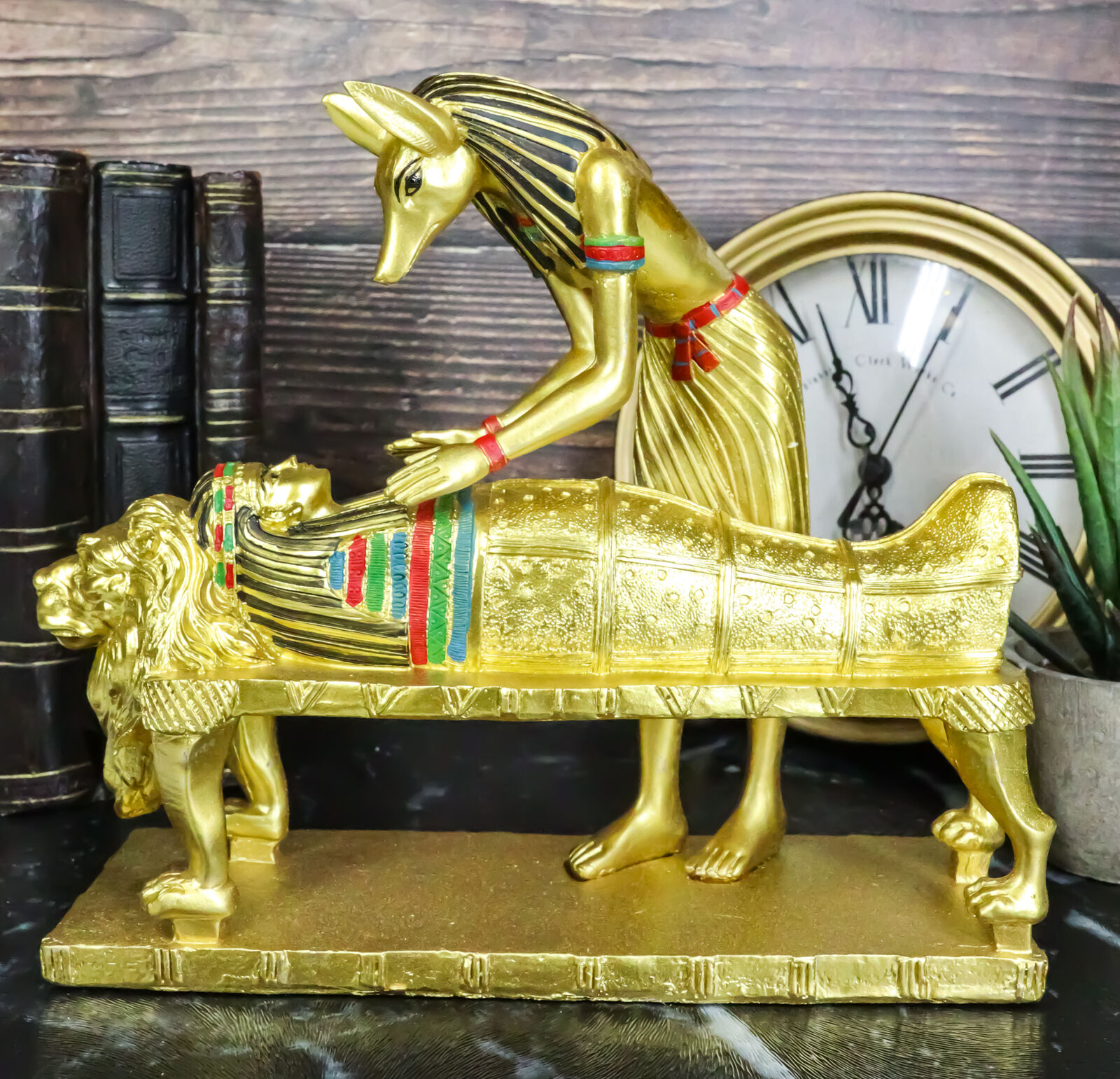The photograph showcases an intricately designed golden Egyptian statue set on a marble table against a background of wood paneling. The central figure is Anubis, the Egyptian god, depicted with a human body and a dog-like head, adorned in traditional markings. Anubis is shown tenderly tending to a female mummy whose casket is ornately decorated with multicolored stripes and a face resembling that of a pharaoh, complete with black-striped details for hair and band. The mummy's casket rests on a bench that features four lion's feet and a lion's head. Surrounding the main figurines, to the left, stand three leather-bound books embellished with gold bindings. On the right side, a small verdant plant and a Roman numeral clock, white with black outlines and encased in a gold frame, add to the décor. This scene forms an exquisite and detailed home decoration that vividly brings ancient Egyptian artistry to life.